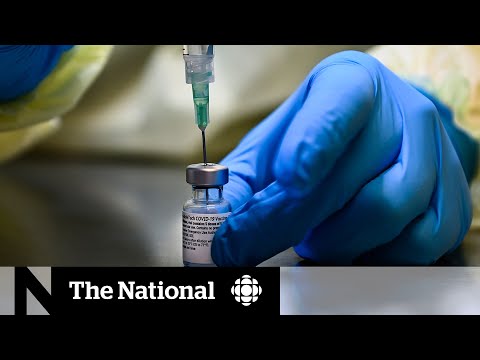The image features a close-up of a gloved hand, adorned in blue medical gloves, holding a vial presumed to contain a vaccine. A syringe with a green-tipped needle is being inserted into the top of the vial. Though the label on the vial is too small and blurry to read, the scene suggests a medical setting, possibly involving someone in white scrubs or a hazmat suit, operating on a plain metal surface. Above and below the main photograph, there are thin black rectangles framing the image. The bottom black rectangle features a decorative opaque white strip, upon which "The National" is displayed in white text. A logo accompanies the text, completing the visually informative and professional appearance of the image.